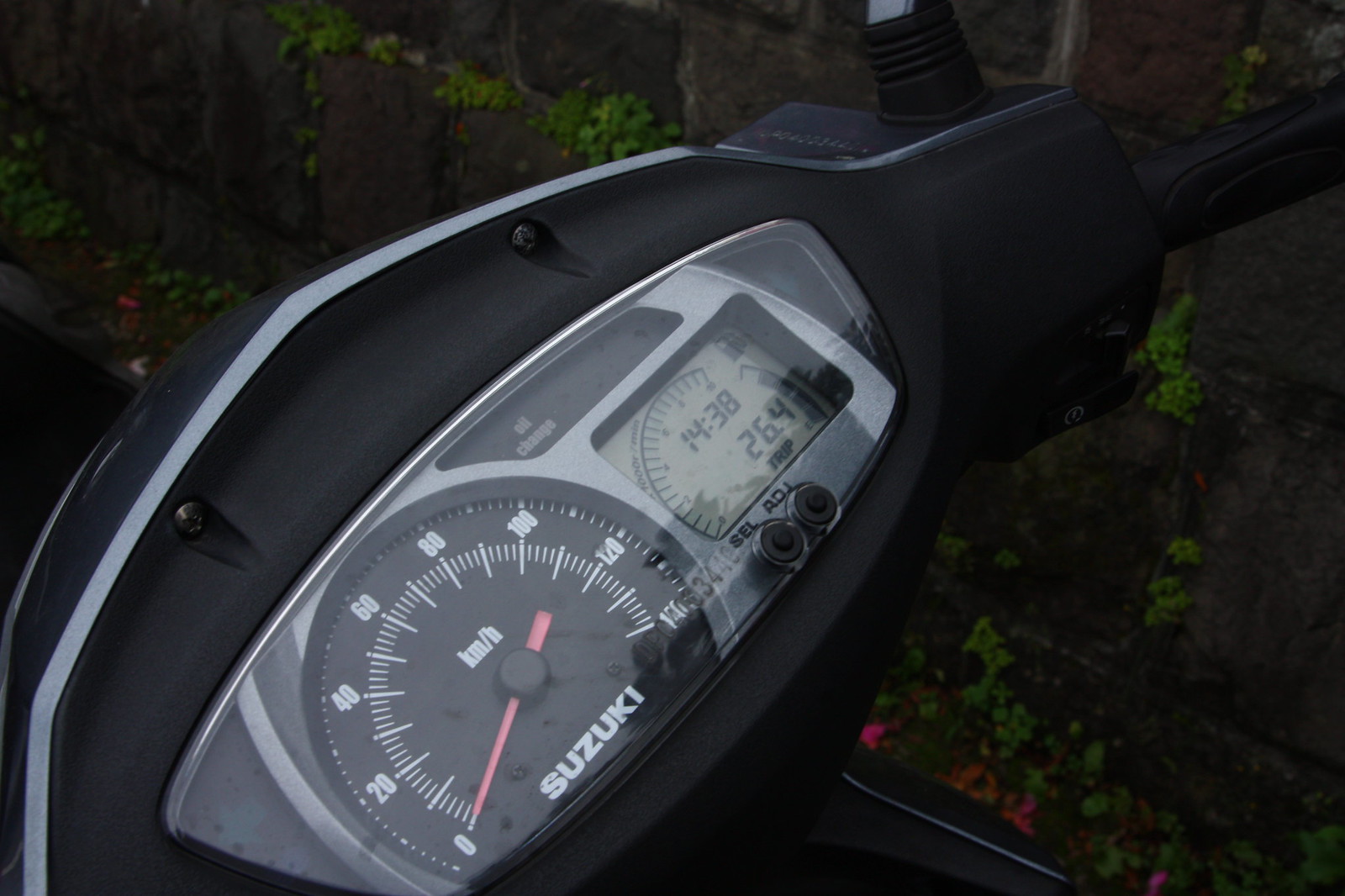This vertical image, taken outdoors, showcases the speedometer and gauge cluster of a Suzuki motorcycle turned at a 45-degree angle. The left side of the bike's control area runs diagonally from the lower left corner to the upper right corner, where part of the handle grip is visible. The gauges are housed in a light gray enclosure secured with a visible bolt.

Dominating the left side is the speedometer, the largest gauge, marked with bold white letters spelling "Suzuki" at the bottom. The speedometer displays the speed in kilometers per hour, with a red needle resting at zero, indicating the bike is currently at rest. 

To the upper right of the speedometer, there is an elongated rectangular indicator panel marked with "oil" and another unreadable word, suggesting an alert related to oil change or oil pressure. Directly below this panel, and to the right of the speedometer, there is another rectangular box displaying multiple readouts: one reads "1438," while another shows "26.4." Two small black circles, likely ignition keyholes or indicator lights, are positioned beneath this gauge.